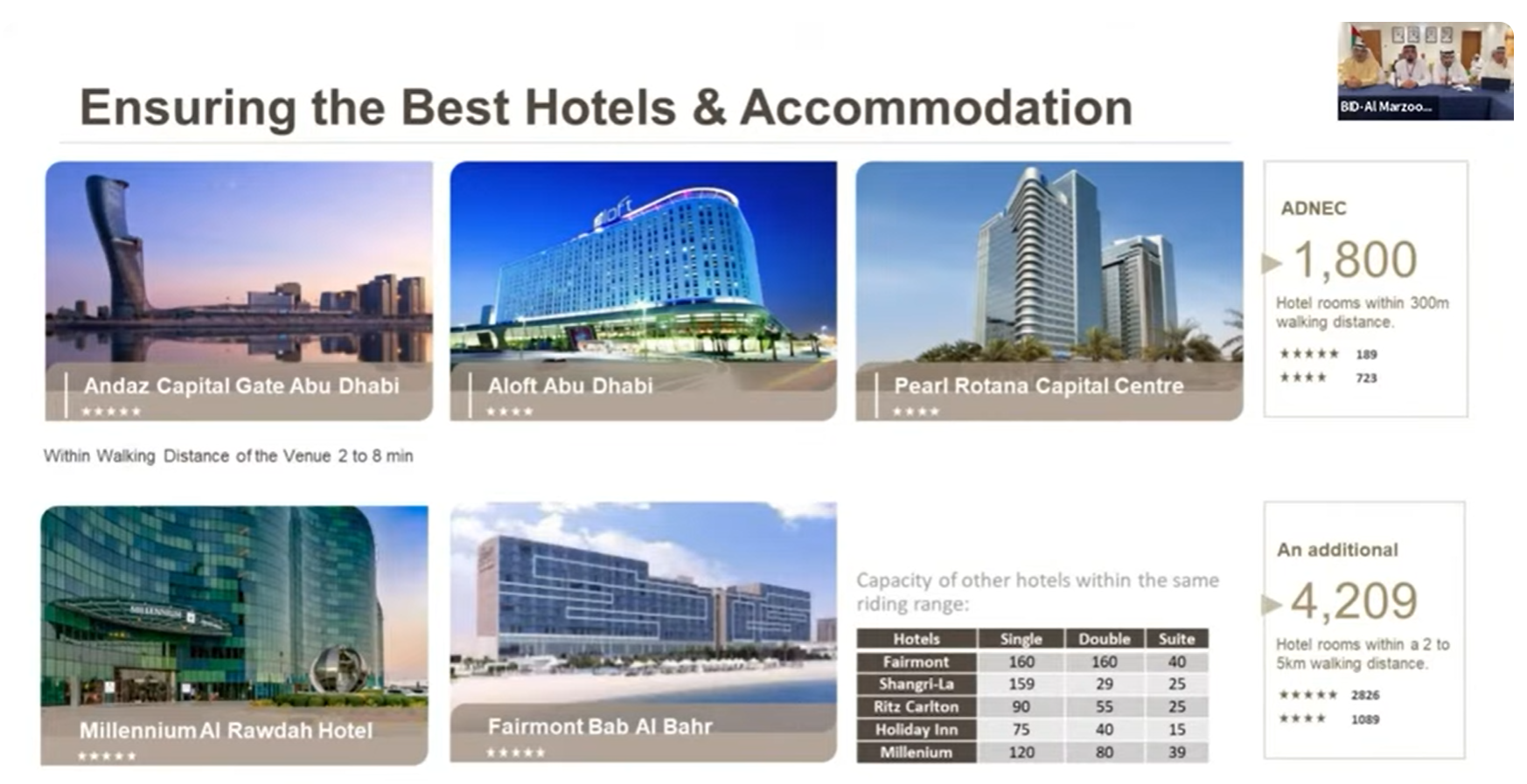**Caption:**  
This detailed screenshot provides an overview of various hotels and accommodations, set against a clean white background. The top of the image features the prominent, bold black heading: "Ensuring the Best Hotels and Accommodations." Directly beneath this, the top row showcases three hotels:

1. **Andes Capital Gate Abu Dhabi**: The leftmost image captures an outdoor view of this hotel across a body of water during sunset or sundown. Notably, it is located within walking distance of the venue, approximately two to eight minutes away.
   
2. **Aloft Abu Dhabi**: The central image on this row depicts an outdoor shot of a tall hotel building that appears almost transparent against the sky. 

3. **Pearl Rotunda Capital Center**: The rightmost image displays an outdoor photograph of this very tall hotel, reminiscent of an office building. It mentions its proximity to ADNEC, being 1800 meters away, with hotel rooms located within 300 meters walking distance.

The subsequent row presents three more hotels:

4. **Millennium Al Rada Hotel**: The first image in this row offers a close-up of the hotel’s front door and some lower floors.
   
5. **Fairmont Bab Al Bar**: The middle image portrays a sprawling, low-rise hotel. Accompanying this is a note about the hotel’s capacity within the same riding range.

Additionally, there is a detailed table of hotel room capacities categorized as single, double, and suite. The text to the right states that there are an additional 4,209 hotel rooms available within a two to five kilometer walking distance.